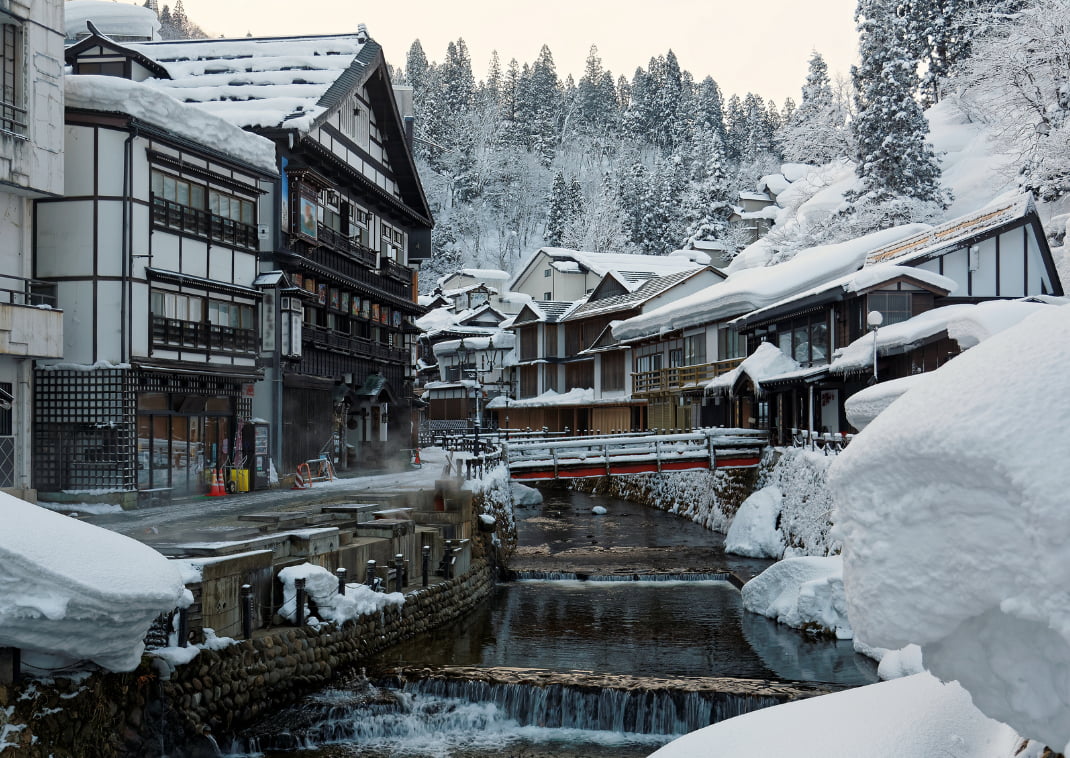In this vivid winter scene, the image captures a quaint village blanketed in snow, nestled at the foot of snow-capped mountains. Central to the picture is a small creek, about 15 feet wide, flowing gently through the town and featuring three small waterfalls, each cascading 2 to 3 feet down. Flanking the creek are charming houses and shops, adorned with thick layers of snow on their roofs and ground, invoking a serene, sleepy village atmosphere. A quaint red and white bridge spans the creek, also cloaked in snow.

The imagery bursts with colors like the pure whites of the snow, vibrant reds and yellows, rich browns, the deep greens of winter forests, and the clear blues of the water—all contributing to the scenic beauty. Trees, heavy with snow, can be seen in the background, adding to the picturesque winter wonderland feel.

This alpine-like town, possibly reminiscent of Switzerland or Bavaria, also bears architectural nuances suggesting it could be in northern Japan, specifically the Hokkaido prefecture. Japanese characters visible in the background further support this setting. The overall composition and the serene atmosphere are indicative of a small, tranquil village somewhere amidst the snowy landscapes of Japan.